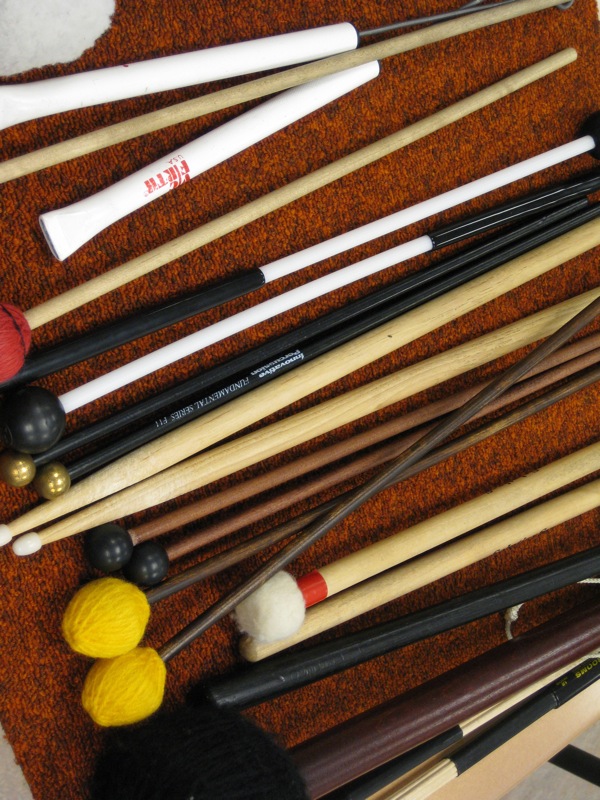The image depicts a collection of various percussion instruments arranged vertically against an orangish-brown, high-fiber carpet. The assortment includes the typical light, pale wooden drumsticks with white plastic tips, commonly used by drummers. Intermixed with these are drum brushes and mallets featuring darker wooden handles. Notably, some of the mallets have strikingly colored ends: yellow, red, and white with the white one appearing particularly cottony. Other items visible include a white whistle with red text and instruments with tan wood handles, including one with an orange fabric ball. Several of the darker wooden sticks are capped with yellow balls, resembling those used in percussion to produce softer sounds. The carpet's texture and color highlight the varied materials and hues of the instruments, creating a homogenous yet detailed visual.